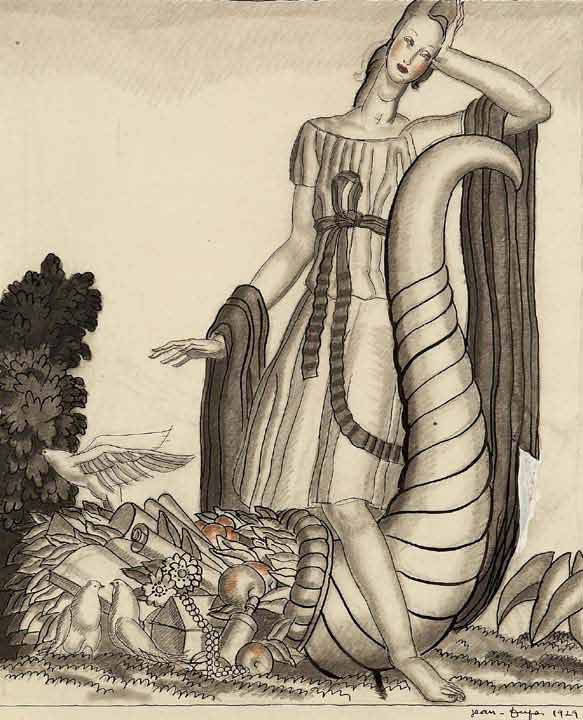This is a detailed black-and-white sketch of a young woman, possibly from an ancient world, depicted as a maiden in a long gown with a pleated skirt and a ribbon tied at her waist. She wears a short-sleeved dress, and over her arms and around her back is a long, dark sash. The woman stands with her left foot in front of, and her right foot behind, a large, ornately crafted cornucopia teeming with fruit, flowers, greenery, and scrolls. Three birds are part of the intricate scene, with two perched on the front and one white bird atop the cornucopia, appearing to eat from a bush on the left side of the image. Her left elbow is resting in a crooked position on the horn of the cornucopia, while her forearm supports her head, which is embellished with a long neck and lips dusted in red. The entire composition rests on a beige piece of paper with a few touches of color, including the orange-red highlights on the fruits within the cornucopia and the woman’s red-painted lips, accentuating the otherwise monochromatic and exquisitely detailed illustration.